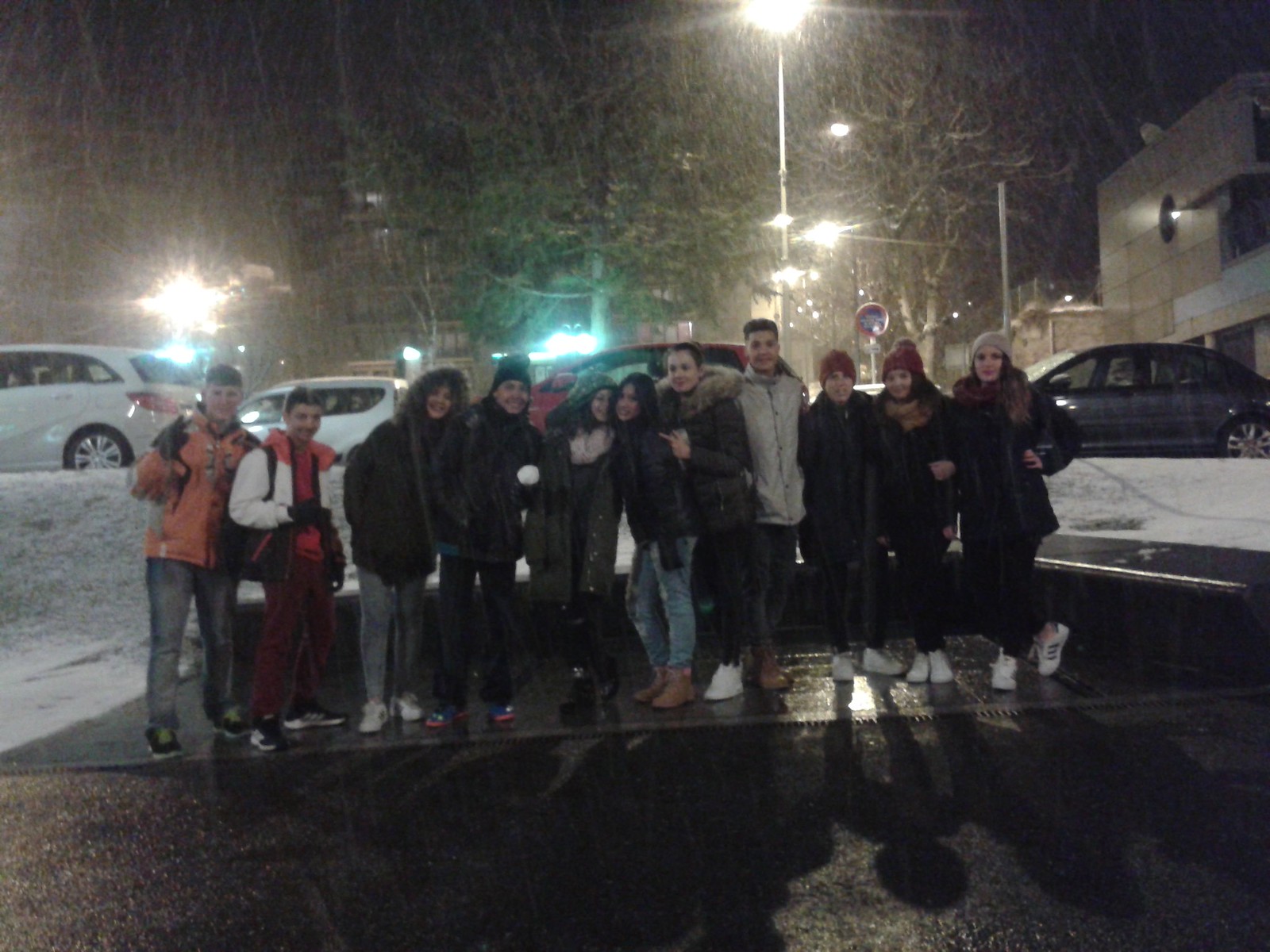The image captures a nighttime outdoor scene featuring approximately 12 young friends standing in a rough line about 10 to 12 feet away from the camera, which might be taken from behind a window, as indicated by the little smears at the top of the picture. The friends, dressed in informal winter attire including coats, hats, gloves, jeans, and black pants, are smiling and appear pleased, with some showing gestures of closeness like putting their arms around each other or leaning against one another. The background reveals a lightly snow-covered landscape with snow particularly visible on the left-hand side and the back right-hand side of the image. The ground they're standing on is wet, possibly from light snow or rain, resembling a cement parking lot. Behind them are several brightly lit cars positioned on a slightly elevated surface, including two white cars, a red car, and a gray car. The setting suggests the group might be gathered in a parking lot, possibly near a school or community center.